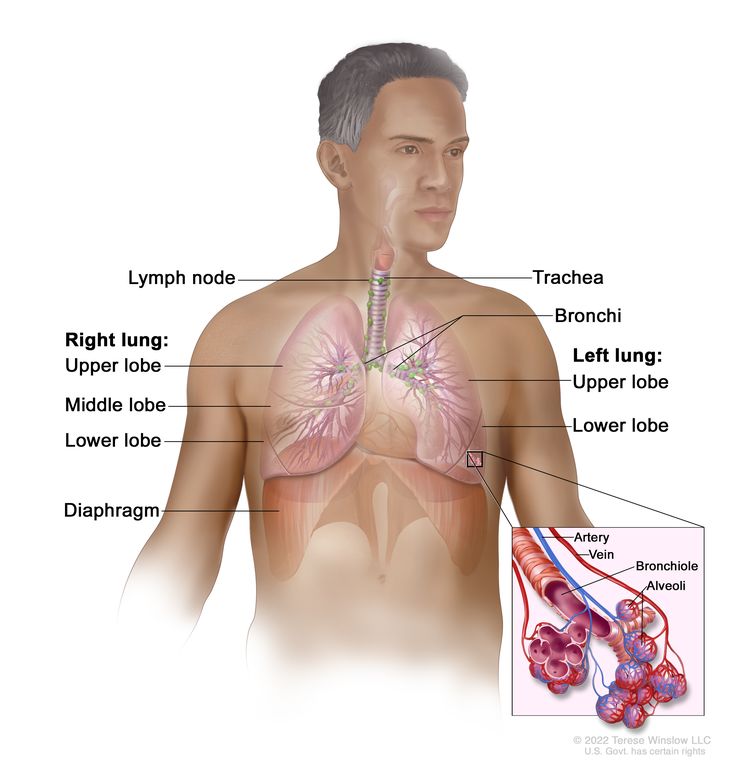This detailed medical illustration depicts an adult man with short black hair, appearing from the top of his head down to just below his belly button, and looking slightly to the left. His skin is beige, almost translucent, revealing the internal structures of his chest. The focus of the diagram is on his respiratory system, including labeled parts such as the trachea, bronchi, and diaphragm. Both lungs are shown in detail, with the left lung divided into the upper and lower lobes, and the right lung divided into the upper, middle, and lower lobes. Additionally, the diagram labels a lymph node. There is an inset close-up view highlighting the intricate details of the artery (red), vein (blue), bronchiole, and alveoli, pointing to the lower left lobe of the lung. The overall image is colored in shades of red, pink, purple, and blue to emphasize the different anatomical features. The man is depicted with his arms outstretched, and there appears to be a marking at the bottom of the illustration, indicating the creation date as 2022 and attributing it to Teresa Winslow LLC, noting certain rights held by the US government.